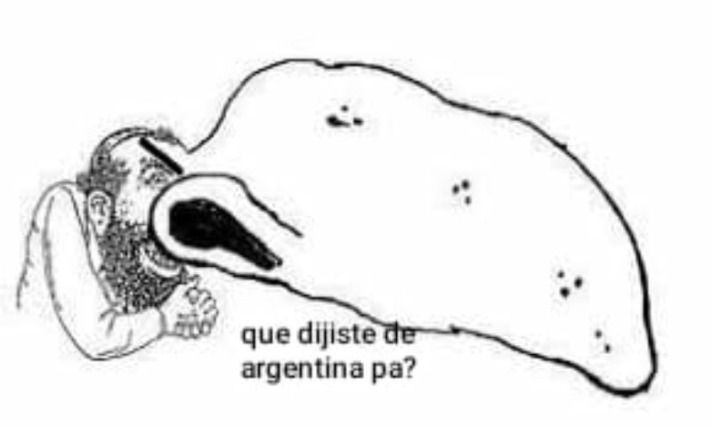The image above is a black and white pencil sketch with a humorous, meme-style caption. It features a cartoonish depiction of a man with an exaggeratedly large nose, which dominates the right side of the image and is marked with crinkles and shadings for emphasis. The man's humongous nose also has a giant, shaded nostril. He has a big beard and sparse hair on top with more growth on the sides, and he is captured with his mouth open, showing his teeth. The man is positioned sitting on an invisible counter with his hands folded or rubbing together. The text in the image repetitively reads, "Que Dieste De Argentina Pa?" which translates loosely to, "Q, did you stay at Argentina, pa?" The overall style of the image suggests it might be propaganda artwork, given its black and white, highly accentuated features.